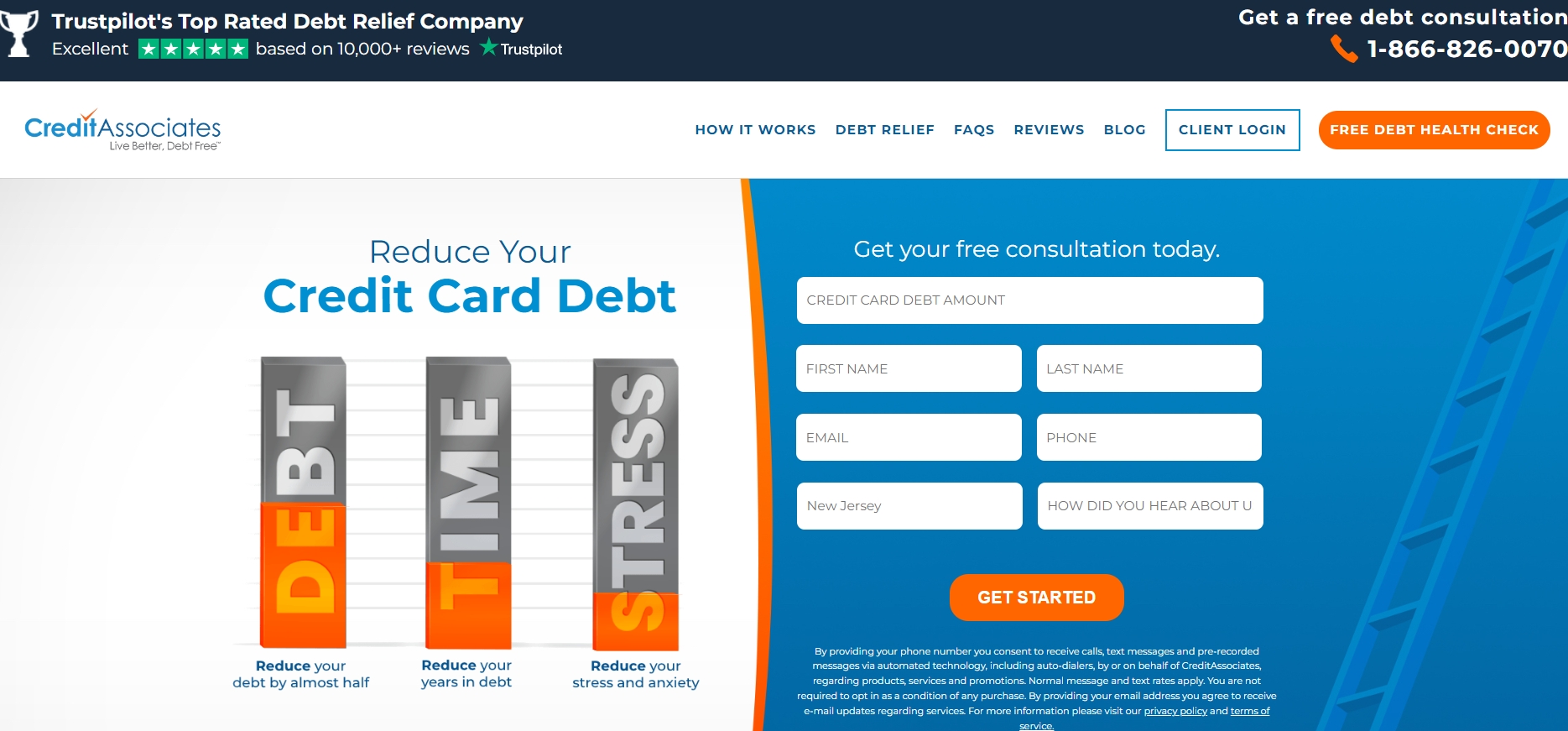The webpage being described is a highly detailed and inviting advertisement for Credit Associates, featured prominently on Trustpilot. The dark banner across the top features "Trustpilot's Top Rated Debt Relief Company" with Trustpilot's logo and motto. To the right, a call-to-action, "Get a Free Debt Consolidation," is followed by a toll-free number: 1-866-826-0070.

Under this, a bold "Excellent" rating is showcased next to five gold stars, with an impressive note of being based on over 10,000 reviews. The word "Trustpilot" emphasizes the credibility of these reviews. Below, the company's name, "Credit Associates," stands out in blue.

Navigation options are clearly presented at the top: "How It Works," "Debt Relief," "FAQs," "Reviews," "Blogs," "Client Login," and "Free Debt Health Check." Below, a clean, user-friendly form encourages visitors to "Get Your Free Consultation Today," asking for details including credit card debt amount, first and last names, email, phone number, location, and a source reference of how they heard about the service. A bright orange "Get Started" button prompts immediate action.

The form is set within a blue box accented by an orange left margin for visual contrast. To the left of the form, three vertically aligned gray boxes— each with a prominent orange initial, "D," "T," and "S"—highlight key benefits: reducing debt by almost half, reducing the years spent in debt, and reducing stress and anxiety. This section is capped by a decisive header, "Reduce Your Credit Card Debt," making the benefits crystal clear.